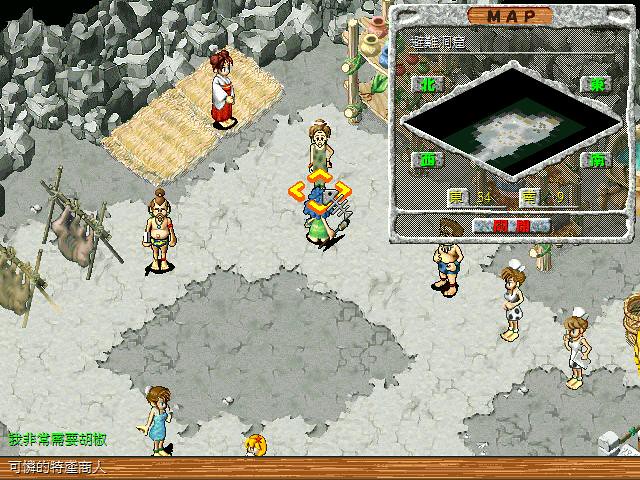In this video game scene, we observe a large concrete floor populated by various characters. Some characters resemble nurses, identifiable by their traditional white hats and blue dresses. Notably, there is a quirky character marked by a small yellow square hovering above its head. The environment also features a shelf lined with an assortment of pottery. Additionally, whole animals are seen roasting on stakes over open fires, adding a dynamic element to the setting. A map is displayed in the upper right corner of the screen, featuring green numbers for navigation. At the bottom, there's a log with two orange stripes, likely indicating progress or status.